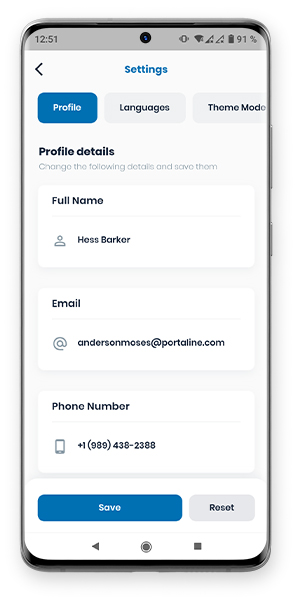This is a detailed color image resembling a mobile phone's user interface, possibly an illustration due to its slightly unrealistic top area. 

At the top, there is a grey band displaying "12:51" on the left side, next to a circular camera sensor in the center. On the right side of the band, there are various icons indicating WiFi connectivity and a 91% battery level. Below the grey band, the interface transitions to a white background. On the left side of this white area, there's a back arrow icon. Centrally, the word "Settings" is prominently written in blue text. 

The screen is organized with three horizontal rectangles beneath the "Settings" title. The left rectangle is blue, labeled "Profiles." The other two rectangles are light grey, labeled "Languages" and "Theme Modes," respectively. 

Further down, there are profile details meant to be edited or updated: the full name "Hes Barker," the email address "andersonmoses@portlean.com," and the phone number "508-438-2288," depicted alongside a small phone icon. 

At the bottom of this section, there are two buttons: a blue button with white text labeled "Save," and a grey button with black text labeled "Reset." 

Lastly, at the very bottom of the screen, there are three navigational icons: a back arrow on the left, a circular home button in the center, and a square icon on the right, reinforcing the impression of a mobile phone interface. This highly detailed depiction, combined with some unrealistic elements at the top, suggests the image might be an artistic illustration rather than a photograph.